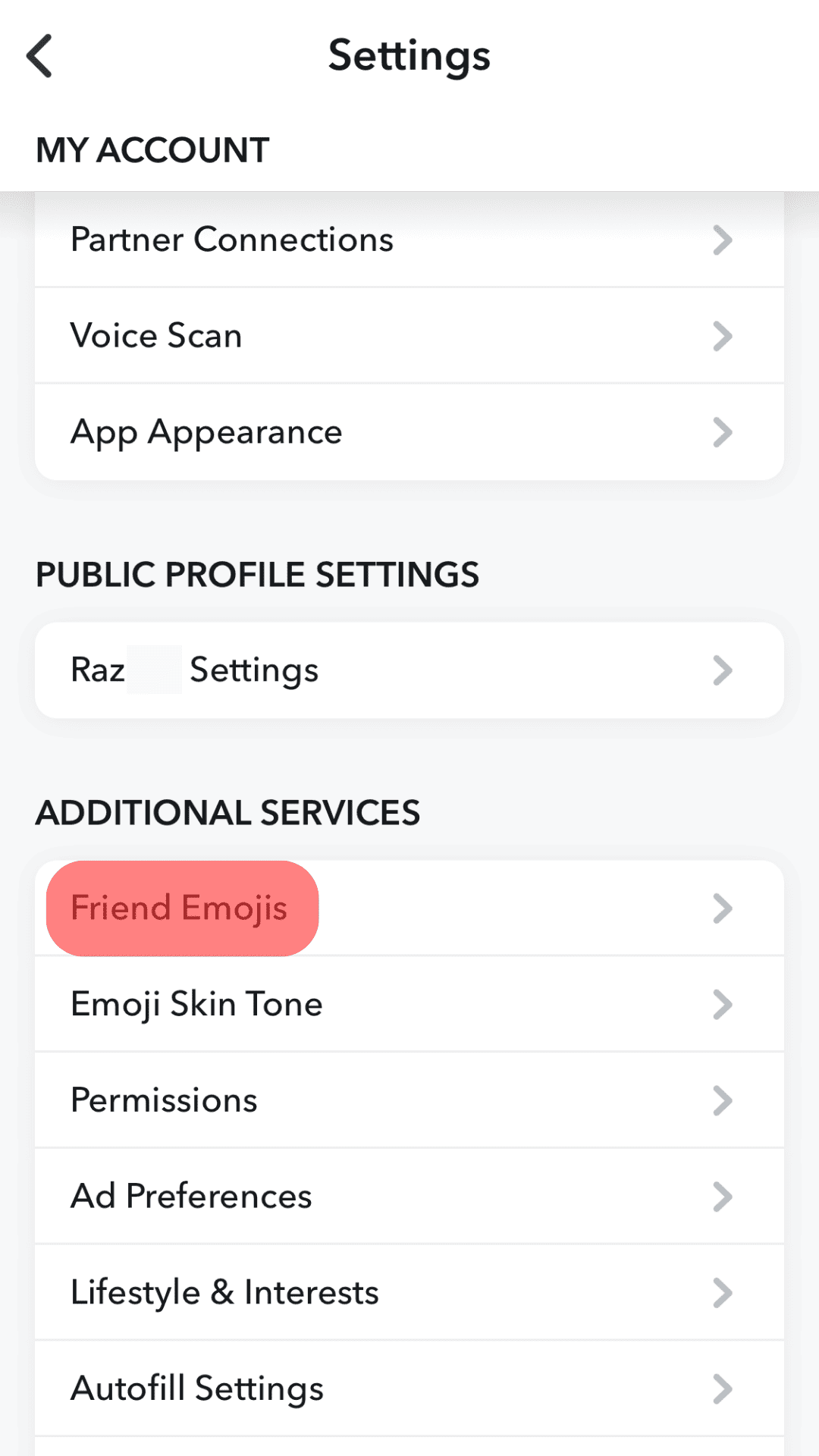This is a detailed and organized caption for the given image:

---

**Screenshot of Settings Menu:**

The screenshot captures the settings page of an application with various options arranged for user customization. At the top center, the word "Settings" is prominently displayed.

- **My Account:**
  - Positioned below a left-justified back arrow.
  - Contains three vertically stacked options:
      1. **Partner Connections** - with a forward-arrow icon indicating additional options.
      2. **Voice Scan** - also featuring a forward-arrow icon.
      3. **App Appearance** - includes a forward-arrow icon.

- **Public Profile Settings:**
  - Contains a section titled "Public Profile Settings."
  - Features "Roz Settings" with an arrow pointing to the right for more options.

- **Additional Services:**
  - This section highlights what's available for user customization:
      1. **Friend Emojis** - displayed in a red box.
      2. **Emoji Skin Tone**
      3. **Permissions**
      4. **Ad Preferences**
      5. **Lifestyle and Interests**
      6. **Autofill Settings**

Each option is accompanied by an icon indicating that further settings can be accessed by clicking or tapping.